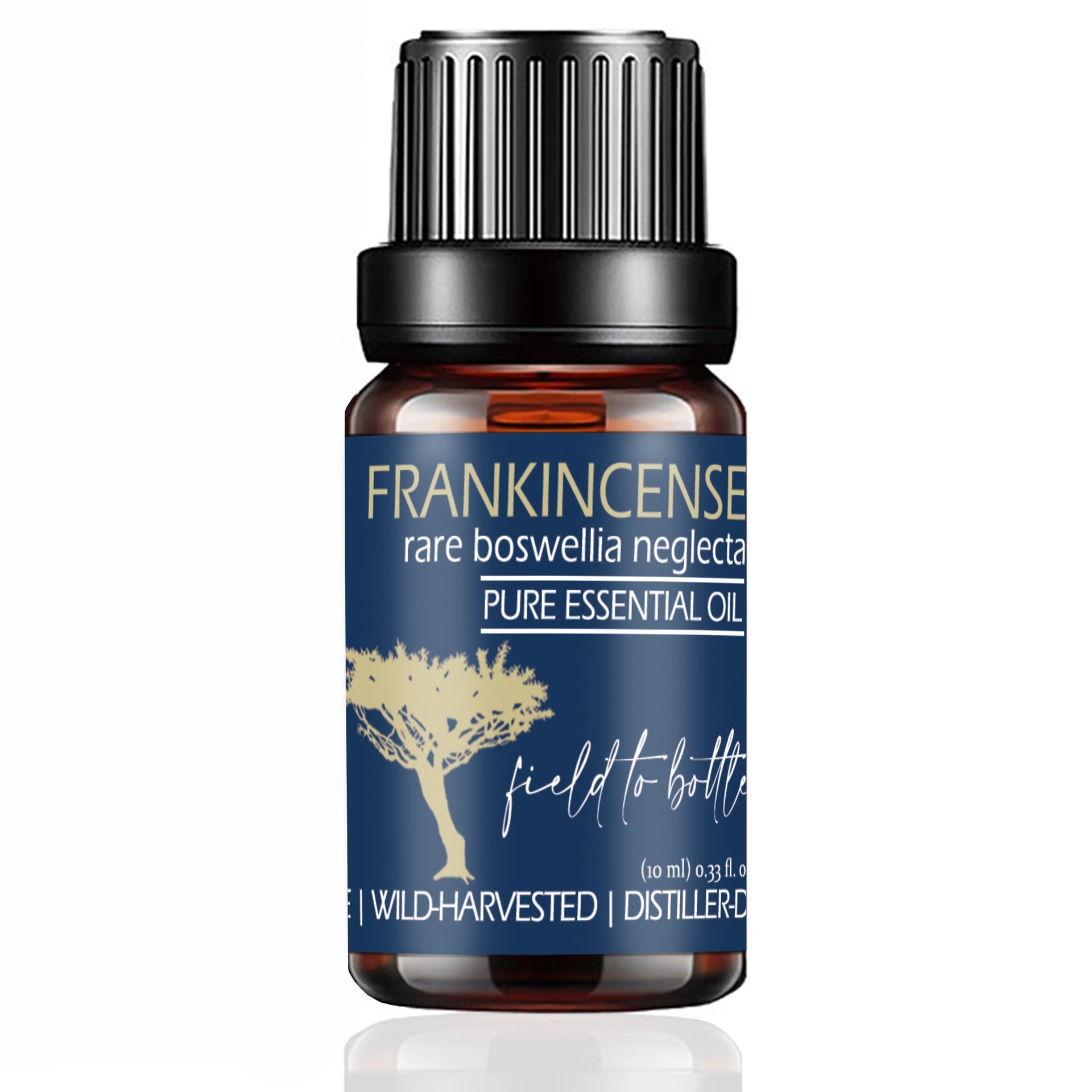The image features a brown bottle with a black ridged cap containing Frankincense Rare Boswellia Neglecta Pure Essential Oil. The label, which is a striking deep blue, is centered on the bottle and includes yellow uppercase text at the top stating "FRANKINCENSE", followed by white lowercase text reading "rare Boswellia neglecta". Below this, framed by lines above and below, it states in white uppercase text "PURE ESSENTIAL OIL". The label also features a gold tree to the left and the phrase "field to bottle" to the right in script. Additionally, at the bottom of the label, it mentions "wild harvest distiller" in white text. This cute, modern-looking bottle holds 10 milliliters or 0.33 fluid ounces of oil, and is set against a purple background. The overall presentation emphasizes the natural, high-quality characteristics of the product.